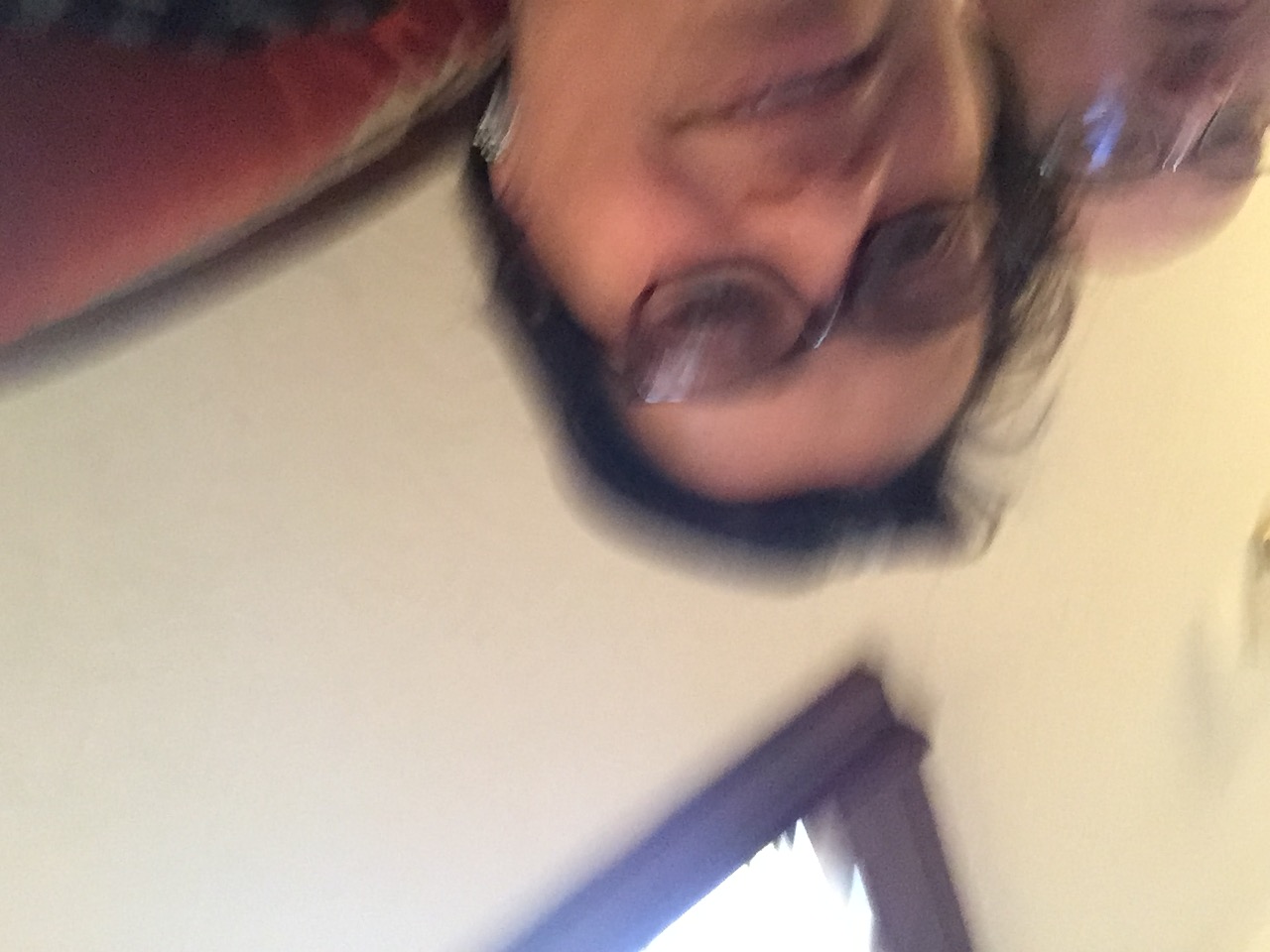In this intimate and candid photograph, a middle-aged couple is seated on a red-cushioned couch in their home. The image, which appears to be a close-up selfie, captures their faces prominently in the frame as they gaze directly into the camera. The woman, possessing short black hair, wears glasses and a noticeable earring in her left ear. Beside her, the bald man, also with glasses, looks at the camera with a neutral expression. Natural light filters through a window above them, gently illuminating the scene but failing to dispel the overall blurriness of the photo. The backdrop reveals a simple setting with white or off-white walls, adding to the cozy and authentic atmosphere of the moment. The woman sports a faint, half-smile, infusing the image with a touch of warmth despite the lack of clarity.